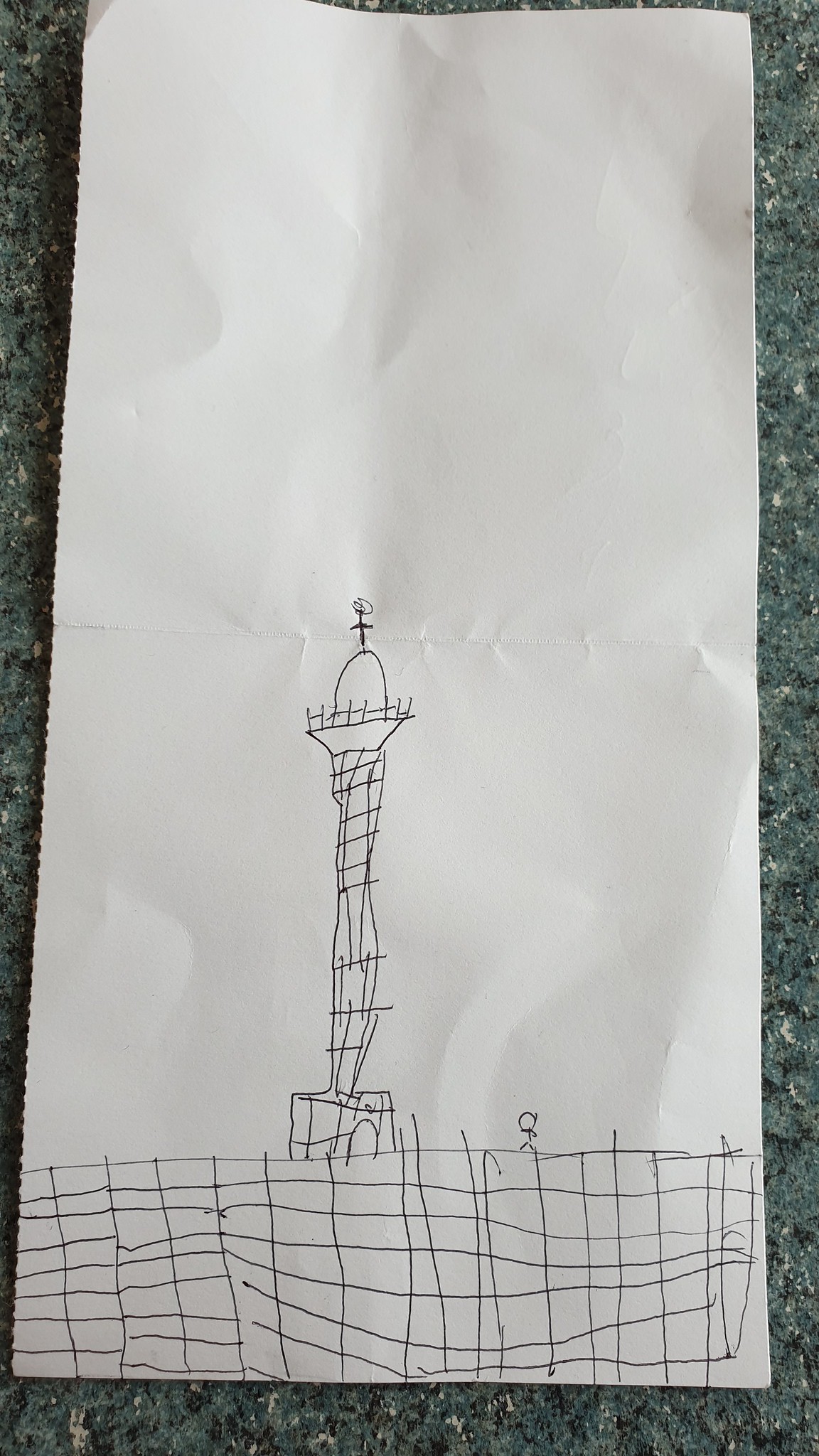A slightly crumpled piece of white paper rests on a grey, granite-like surface, showing signs of wear at the top and bottom edges. The paper features a sketch, reminiscent of a child's drawing, illustrating a stick figure with a large round head. The scene depicts a structure, seemingly a wall marked out in grid squares, next to a tower perched on a plinth. The tower extends upward to a flared terrace with a railing. At the pinnacle of the tower is a cupola, crowned with a cross encircled by a ball. The simplistic and rough nature of the drawing contributes to its childlike charm.